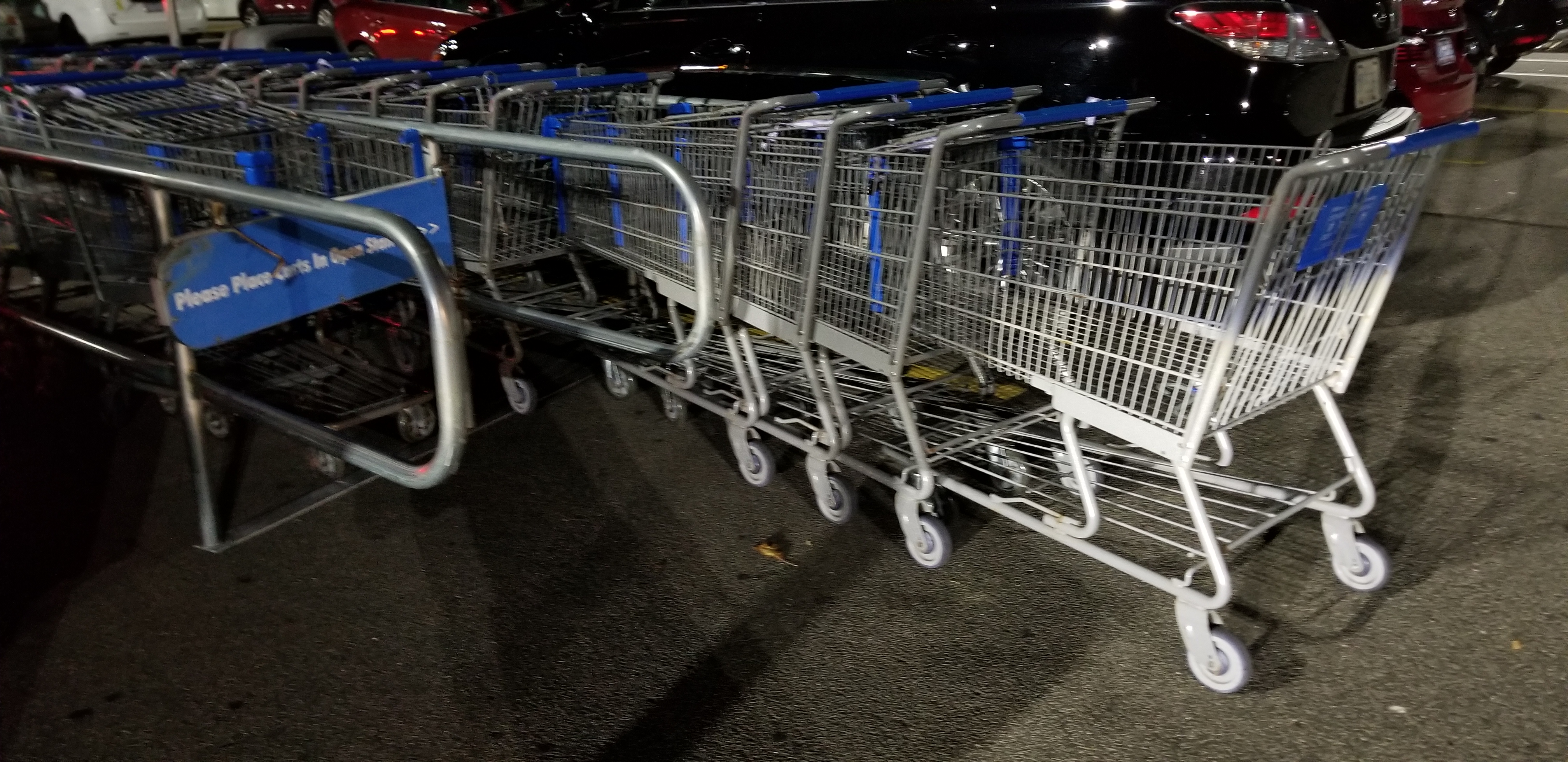The image shows an assortment of Walmart shopping carts, easily identifiable by their light gray frames and signature blue handles, stacked haphazardly within a metal shopping cart return area located in a parking lot. The capacity of the return area is overwhelmed, causing some carts to spill out onto the dark gray asphalt pavement below. A blue sign is visible on the right, partially obscured by a pole, with legible text instructing to "please place carts in open something." In the background, several cars are parked, including a prominent black car with red brake lights illuminated and a red car visible just behind it. Scattered leaves and shadows are cast across the scene, indicating it is nighttime. Silver metal bars frame the area, adding to the organized yet congested nature of the shopping cart return.